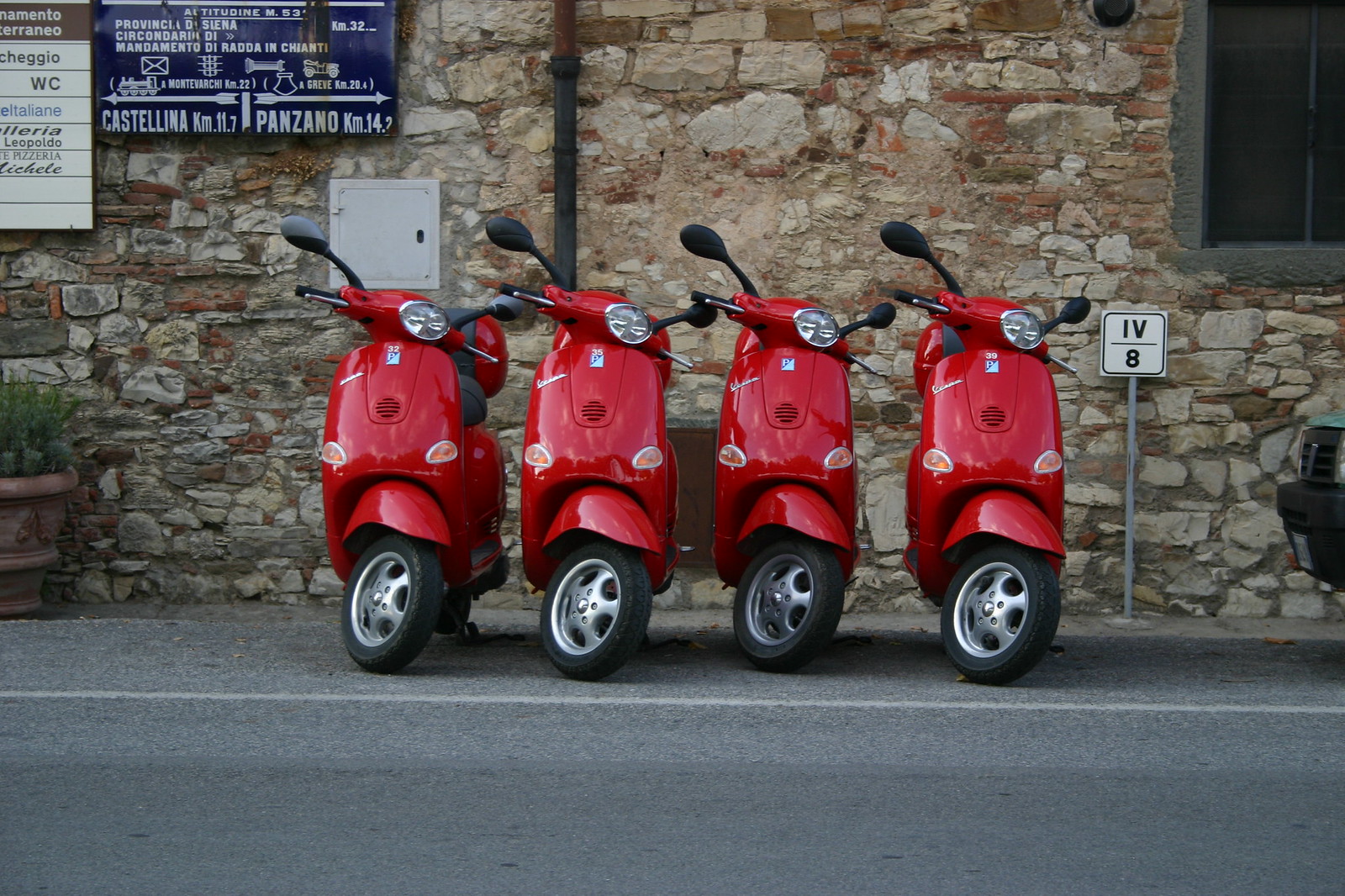In this photo, four brand-new red Vespas are parked on the side of a paved road, neatly lined up with their fronts facing outward towards the street. They are situated to the left of a white line that marks the edge of the road. These mopeds are parked against the stone facade of an old-fashioned building made of white stones, with a reddish-brown coating between the stones. Above the scooters, there is a small white sign on a pole that reads "IV" over "8". To the left of this sign, a gray-trimmed window is partially visible. Additionally, an electric panel box can be seen mounted on the wall behind the mopeds, alongside a terracotta flower pot with some greenery.

The upper left corner of the image features two more signs mounted on the stone wall. The first is a blue sign with white writing indicating directions: "Ponzano, 14 kilometers" to the right, and "Castellina, 11 kilometers" to the left, suggesting the scene is set in an Italian locale. The second sign, white and tan, provides information about the building's amenities, including the presence of a WC (water closet) and various businesses.